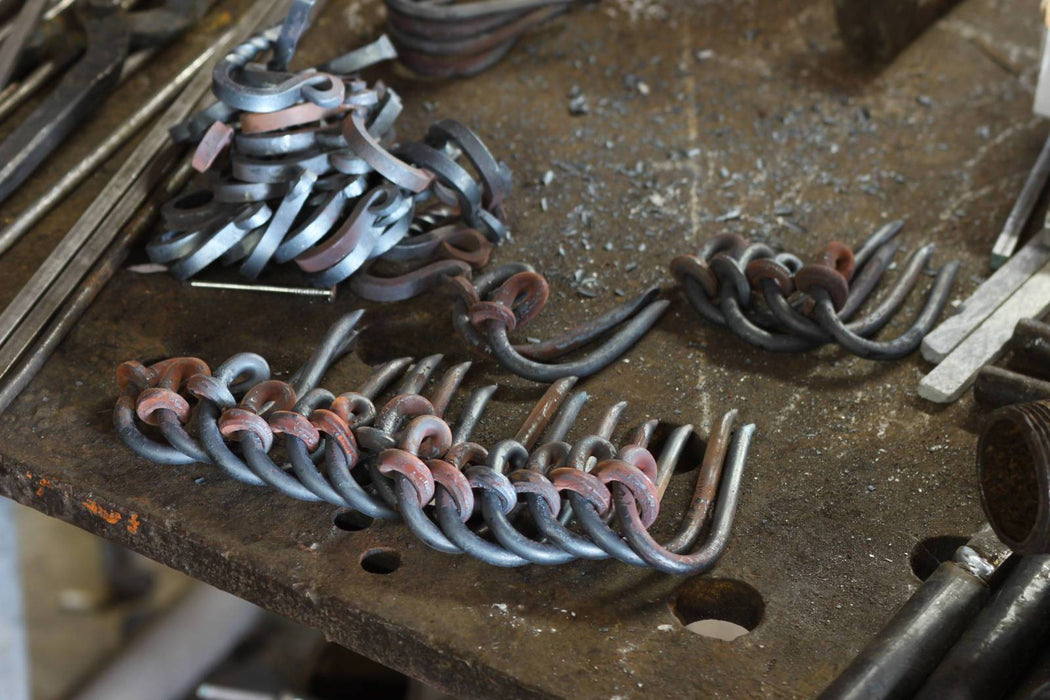This image captures a close-up of a worn, heavily used metal workbench situated in a dimly lit workshop. The table, showing signs of years of diligent metalwork, is strewn with metal shavings. In the foreground, the table features a set of drilled holes—two smaller ones on the left and larger quarter-sized ones on the right. Scattered across the table are various metal rods and bars, particularly noticeable in the lower corners of the image. The focal point is a collection of silver metal hooks meticulously arranged both horizontally and in a pile towards the top left of the photo. These hooks are bundled together by distinctive pink or red bands, akin to rubber bands. Behind the main arrangement, another heap of hooks lies, mostly silver with a few bearing pink and gray hues. The entire scene is set against the backdrop of an industrial environment, with parts of the table’s leg and a crossbar just visible, reinforcing the setting of a seasoned craftsman's workspace.